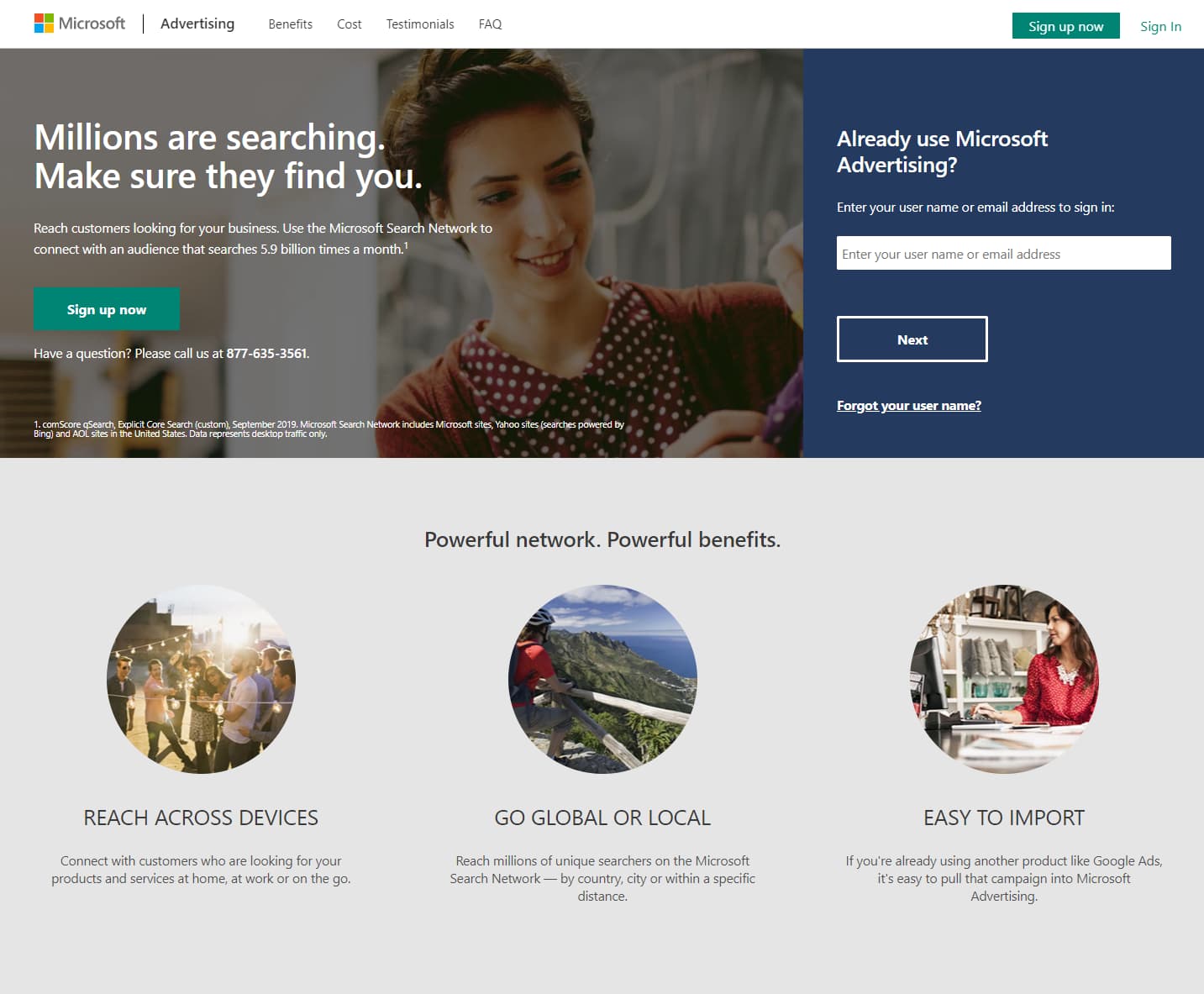**Screenshot of Microsoft Advertising Website:**

The screenshot depicts the Microsoft Advertising home page, featuring a clean, white background with the Microsoft logo—a combination of four squares in red, green, blue, and yellow—positioned at the top left. In bold and selected, "Advertising" is highlighted alongside other navigation options including Benefits, Costs, Testimonials, and FAQ.

On the top right, the page features a green button with white text urging users to "Sign Up Now," beside a blue "Sign In" option. Below, a striking image of a young woman in her early 20s, wearing a polka-dotted shirt under red overalls, captures attention as she examines a dress. Accompanied by the tagline, "Millions are searching. Make sure they find you," the text is presented in white against the background.

Further down, an invitation encourages users to "Reach customers looking for business" by utilizing the Microsoft Search Network's extensive reach, which boasts 5.9 billion monthly interactions. A green "Sign Up Now" button with white text stands prominently below this information. 

For inquiries, a contact number, 877-635-3561, is provided. Small legal text can be seen at the bottom, although it is difficult to read in this context.

Additionally, on the right side, there's a section for existing users to sign in. The prompt states, "Already use Microsoft Advertising? Enter your username or email address to sign in," followed by input fields and a "Next" button, as well as a "Forgot your username?" option.

The lower portion of the page emphasizes the benefits of reaching across different devices with varied illustrative images: a group of people partying, an individual looking over a mountain bridge, and a woman seemingly working in a clothing store. Although text beneath these images is partially obscured, the message relayed is one of powerful networking and significant business advantages through Microsoft's platform.